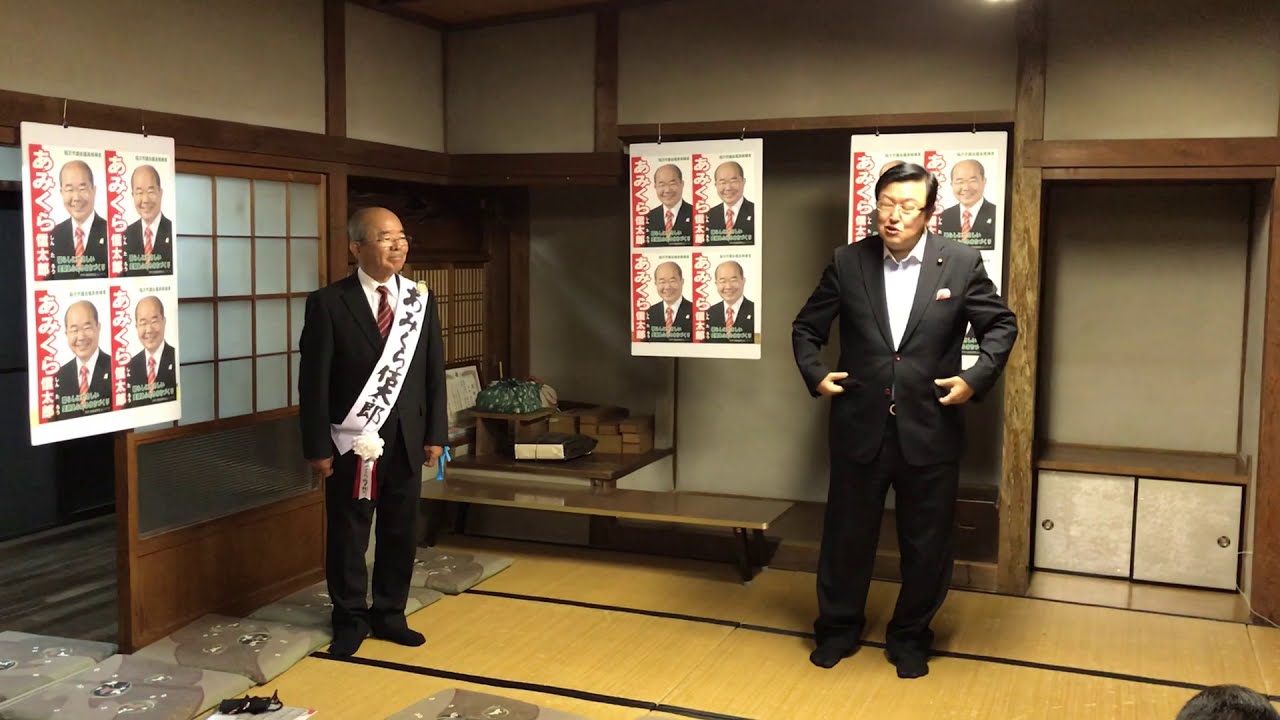In the image, two men are standing in an indoor setting on a mat without wearing shoes, only socks. Both men are dressed in black suits with white shirts. The man on the left stands out with a red striped tie, a bald head with some hair on the sides, spectacles, and a white sash with black Chinese or Japanese writing draped across his chest. He appears older and is the focus of several posters on the walls behind him, suggesting he is being honored or facilitated. The other man, standing slightly apart, has dark hair and no tie. His hands are near his waist, and he appears to be speaking, with his mouth open and eyes closed. The room features white, tan, and brown walls with various pictures of the older man, possibly indicating a campaign or office-related setting. There are also low-height tables with items on them, shelves, cabinets, and cushions arranged on the floor, giving a sense of a traditional, perhaps Japanese-style interior.